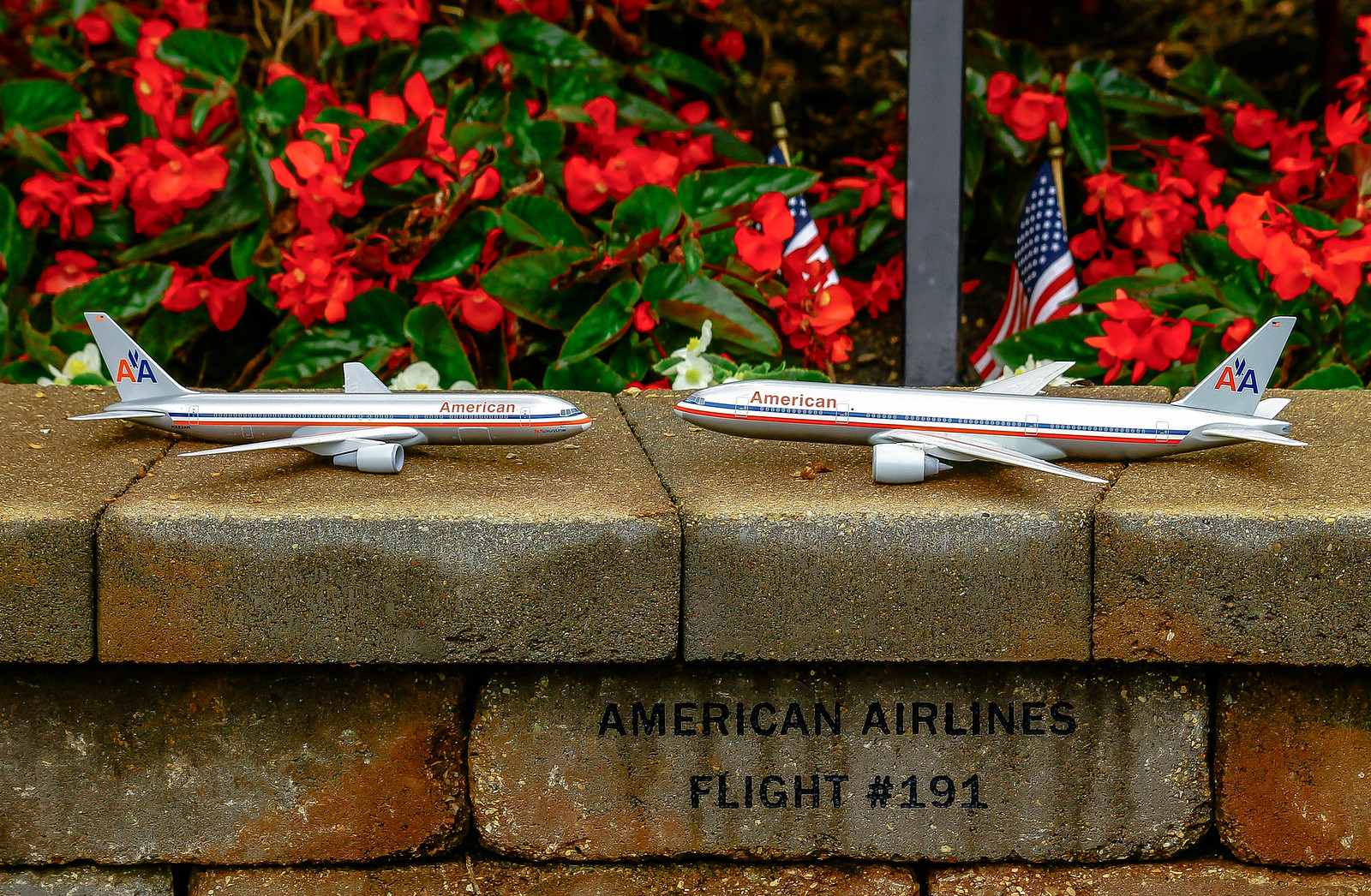The image captures a memorial dedicated to American Airlines Flight 191, featuring two white, miniature airplanes facing each other atop a stone ledge. Each airplane has "American" inscribed on its side, along with the American Airlines logo on the tail - a red and blue capital "A" with wings in the middle. Carved into one of the bricks beneath the ledge are the words "American Airlines Flight 191." Behind the ledge stand two small American flags flanking a metal pole, creating a patriotic backdrop. Surrounding the base of the memorial is a flower bed filled with bright red begonias, displaying their distinctive waxy leaves and angel-like wings. The combination of these elements creates a heartfelt and vivid tribute.